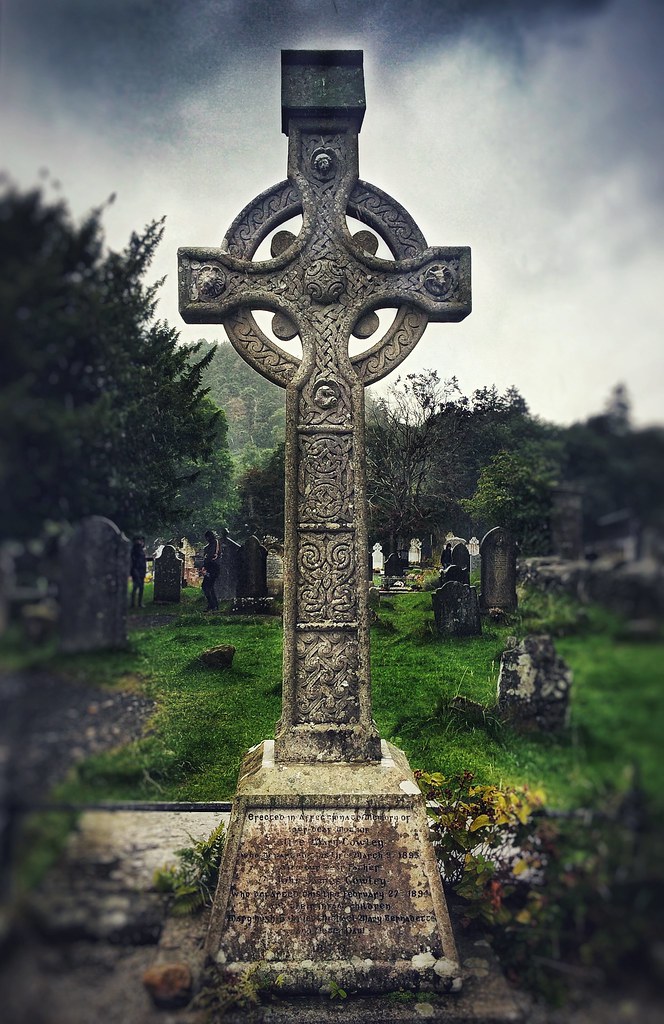This detailed photograph captures an old cemetery under a dark, cloudy sky, suggesting an impending storm. The foreground is dominated by a large, imposing headstone sculpted into a concrete cross with a decorative circle encircling its upper section. The weathered tombstone shows signs of age, including moss, rust, and dirt, obscuring its inscription. Ornate designs are faintly visible on the cross. Surrounding this headstone are yellow and white flowers, contributing a touch of color to an otherwise somber scene. The grave site itself appears untended, with overgrown grass and headstones that have fallen or tilted. The background reveals numerous smaller, varied tombstones dispersed across the green, unmanicured cemetery grounds, along with tall trees that frame the scene. Two individuals can be seen near a grave, adding a human element to the tranquil, if somewhat eerie, atmosphere. The sides of the image are blurred, lending a misty quality to the distant, densely wooded backdrop.